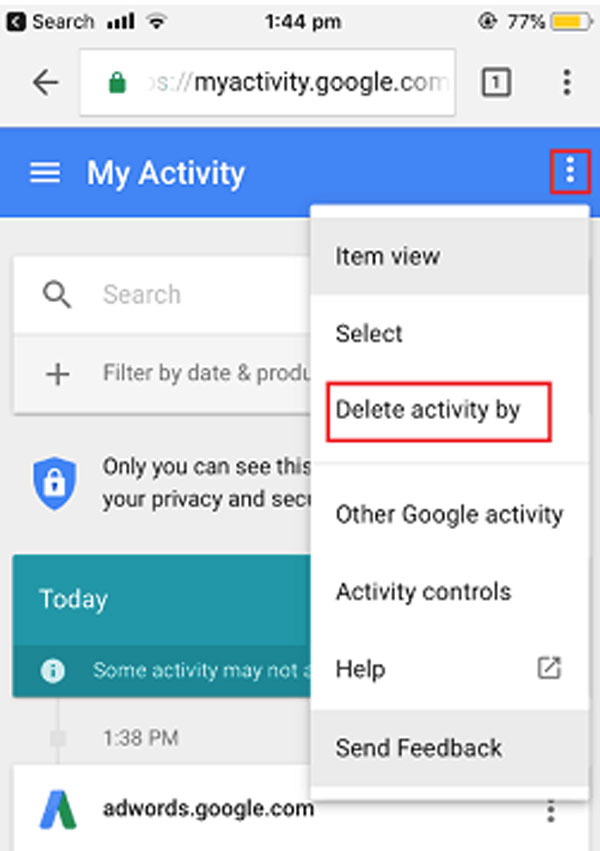This is a detailed screenshot taken at 1:44 PM, showcasing a device with a 77% battery level. At the top of the screen, there is a left-facing arrow and a secure green lock icon, indicating a safe browsing session. The URL displayed is "myactivity.google.com," accompanied by a badge with the number 1 in a square, and three vertical dots to the right, possibly for additional options.

The primary tab visible is labeled "My Activity," featuring various sections, including "Item view," "Select Delete Activity By," "Other Google Activity," "Activity Controls," and "Help." The "Send Feedback" option is distinctly highlighted, suggesting it has been recently interacted with.

In the middle of the screen, there's a timestamp indicating activity from 1:38 PM, specifically for the website "www.adwords.google.com." This detailed view allows the user to manage or review their Google activity with precision.